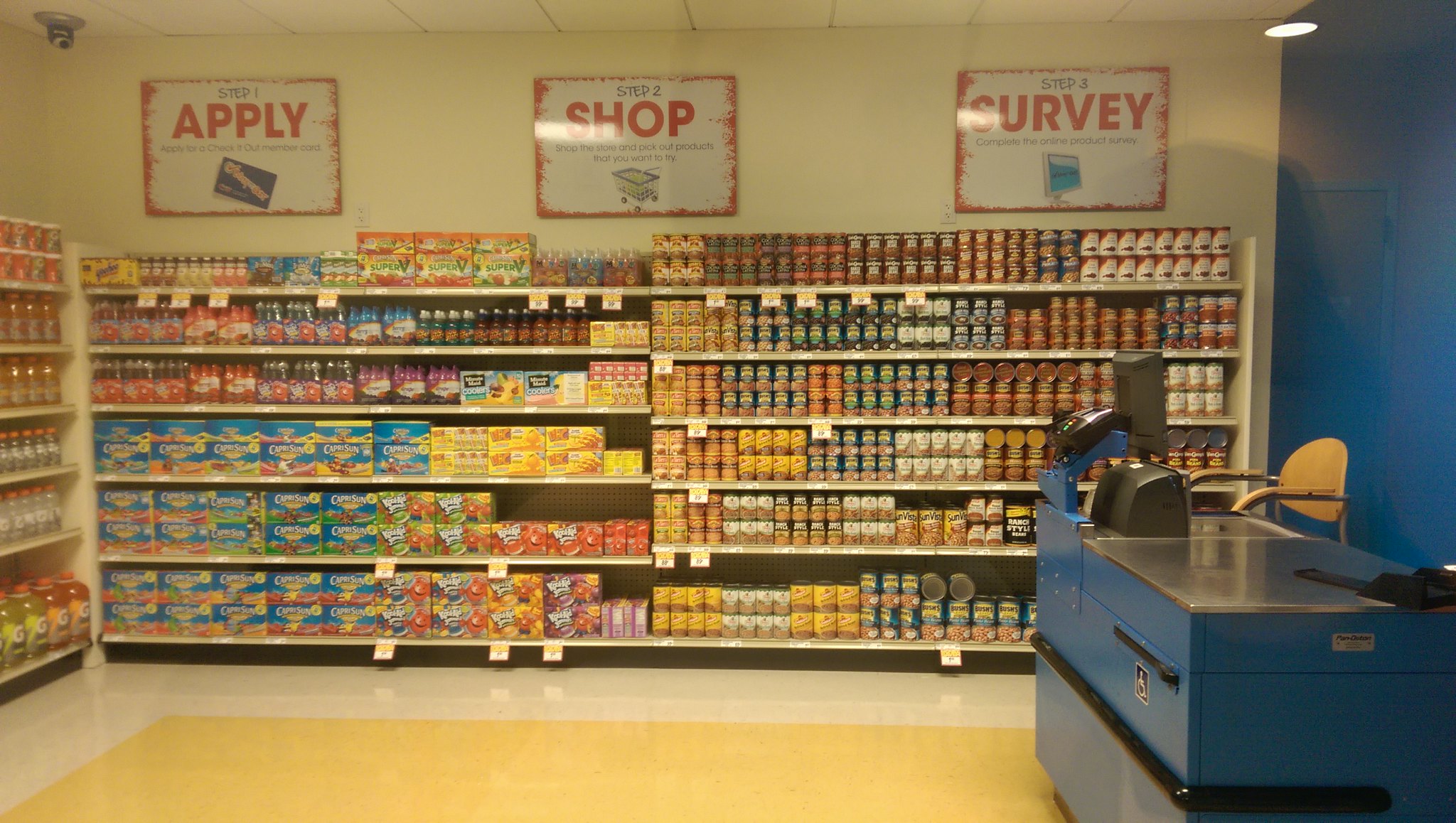This image depicts a well-stocked grocery store with a meticulous and organized setup. Dominating the scene is a large wall display filled with an extensive variety of canned goods. The shelves are organized in a visually appealing manner, with colorful labels creating a vibrant array from top to bottom--red, brown, white labels, yellow on the second shelf likely indicating pickles, green labels, and other yellow items. Above these shelves are three rectangular signs with white backgrounds and red print, stating: "Step One: Apply," "Step Two: Shop," and "Step Three: Survey," sequentially from left to right. 

To the left of this shelving unit, there is an assortment of beverages, including familiar brands such as Capri Sun, Minute Maid, and Kool-Aid. In the front right of the image stands a checkout counter, notable for its blue color and handicap sticker, suggesting an inclusive design. The counter appears rustic and simple, without a conveyor belt, hinting at either an older style or a non-U.S. locale. Just beside this counter, an additional shelving unit is visible, likely housing more bottled juices. The overall setting suggests a warm, inviting, and efficiently organized store environment.